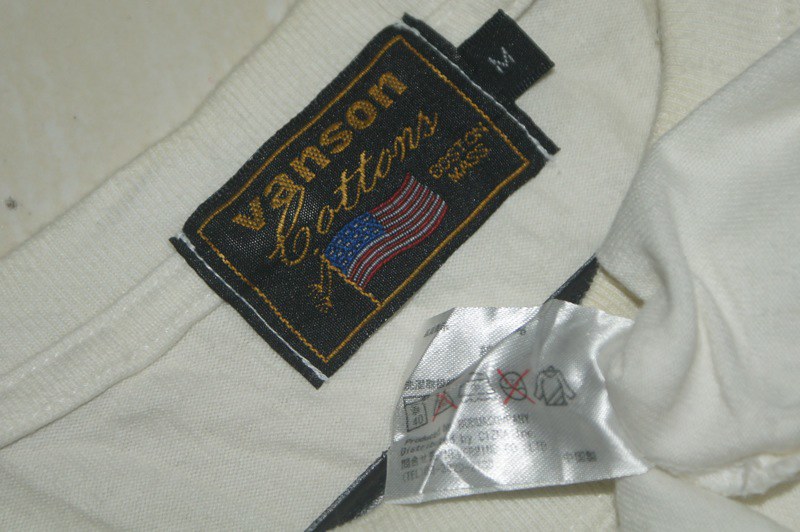This is a detailed close-up photograph of the inside neckline of a white, or slightly off-white, crew neck t-shirt or light sweatshirt. The black label, sewn into the inner neck hem, prominently features the brand name "Vanson Cottons" in gold or bronzy-colored thread. Adjacent to the brand name is an American flag with a golden flagpole. Below the flag, the label reads "Boston, Massachusetts." On the right side of this main label, there's a brown tab indicating the medium size with an "M" in white. Beneath this, a shiny satin care label provides washing and drying instructions, partially visible with black writing and red X marks. The photograph also hints at additional white material, possibly another garment, adding to the layered appearance of the image.